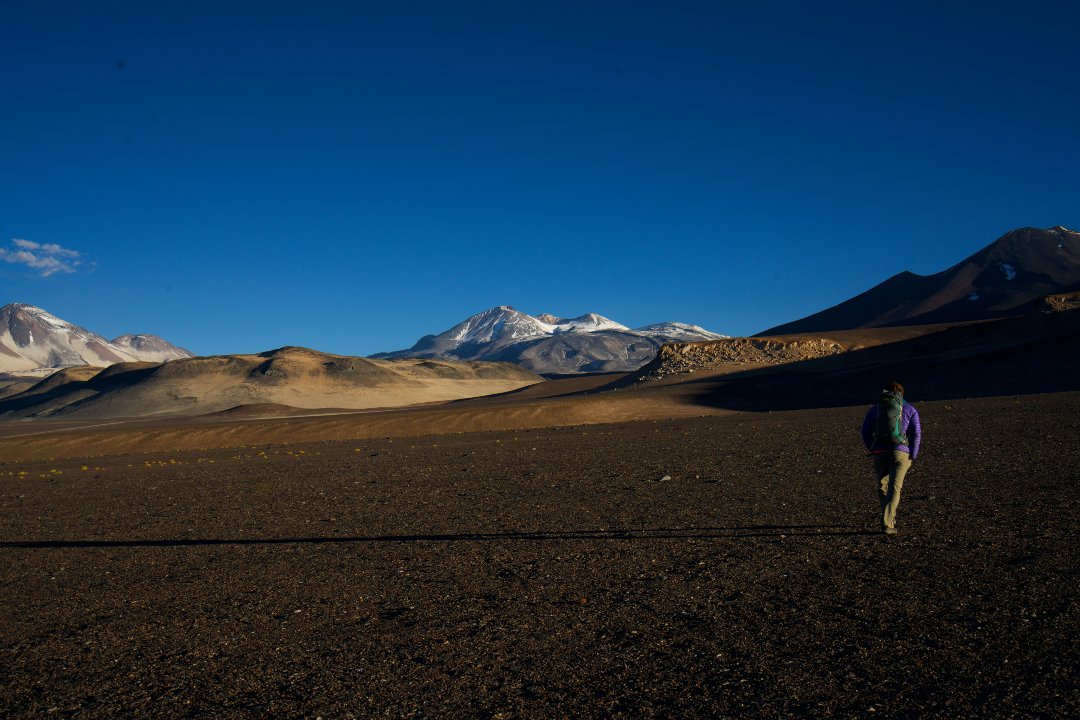In this detailed photograph taken outdoors, likely nearing sunset, a young person, with their back to the camera, is depicted walking in a rugged, barren, mountainous area. The clear, blue sky in the distance features a small cluster of white clouds towards the upper left, transitioning to a deeper blue at the top of the image. Snow-capped mountains dominate the middle of the picture with additional peaks visible on both the left and right edges. The foreground consists of smooth brown dirt and sand that gradually lightens as it recedes toward the distant mountains. Positioned on the right side of the image, the person is clad in a long-sleeved purple jacket, khaki pants, and a large gray and blue backpack. They are walking up the hill with hands in their pockets, casting a long, narrow shadow that stretches leftward across the frame. The photograph, rectangular in shape, measures approximately six inches wide and four inches high, capturing the serene and stark beauty of this expansive landscape.